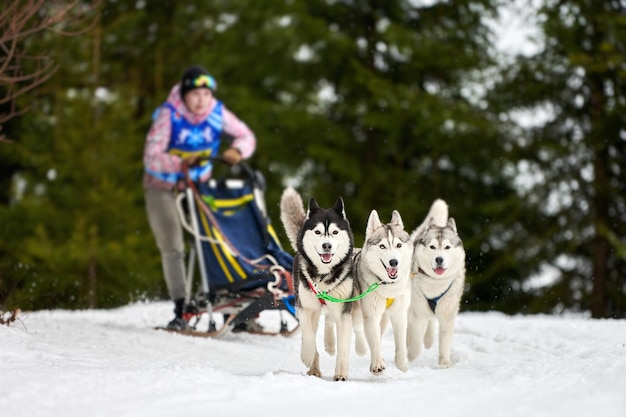In this captivating professional outdoor photograph, a woman, wearing reflective ski goggles, a beanie, a pink and white shirt with a blue vest, and gray pants, is being pulled on a sled by three exuberant Huskies through a snowy forest. The scene is filled with towering trees, while a thick blanket of snow covers the ground, suggesting a recent snowstorm despite the branches being bare. The Huskies, harnessed and lined up energetically side-by-side, seem young and lively. On the left is a Husky with striking white and black fur, while the two on the right are predominantly white with patches of gray. Their joyful expressions capture the essence of the moment, highlighting the excitement and sheer joy of dashing through the snow in what appears to be a race. The sled, resembling a cross between a snow ski and a stroller, glides swiftly behind them, carrying the blurred figure of the woman who's clearly reveling in the adventure.